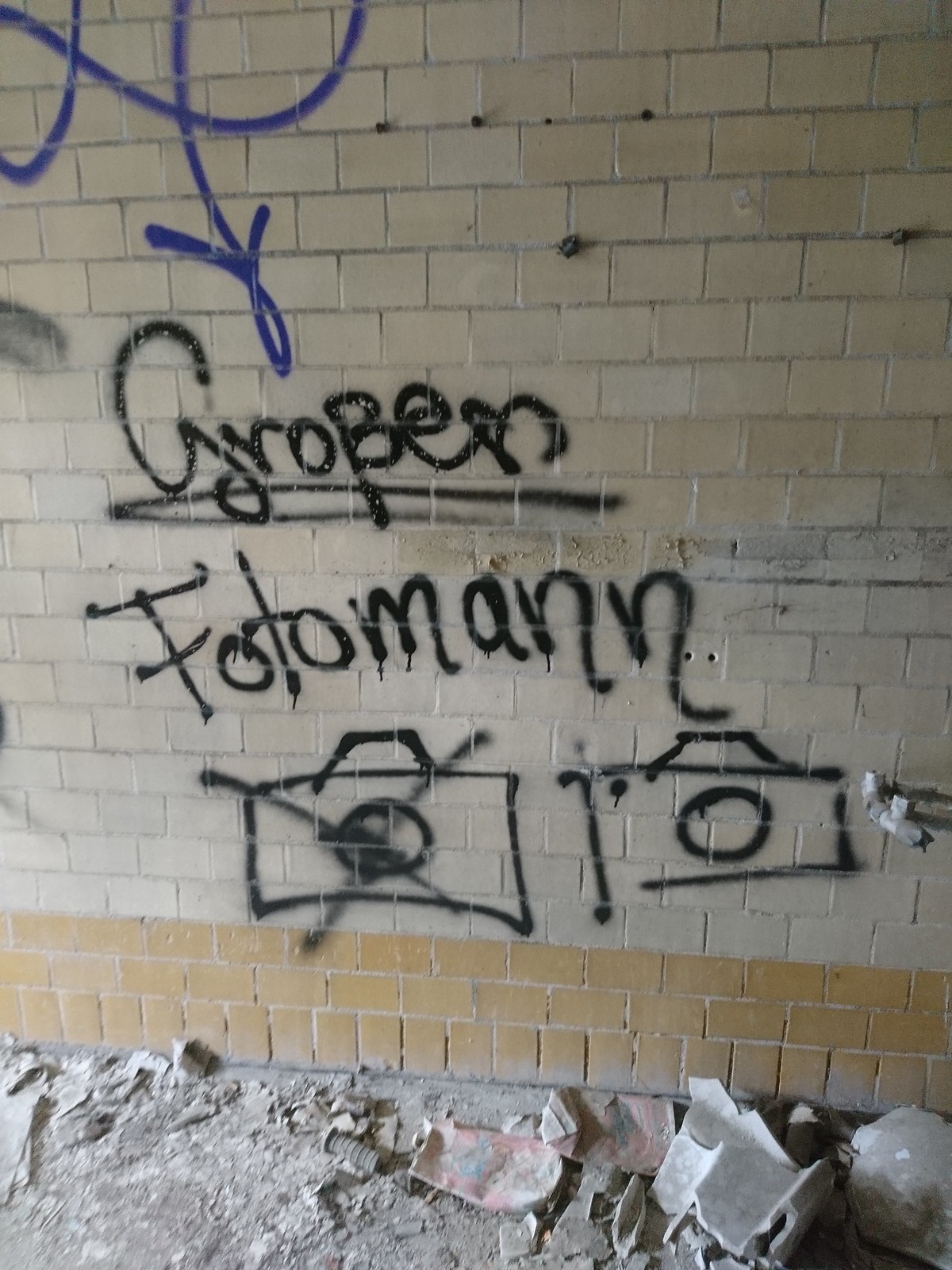The image depicts an old, discolored brick wall segmented into three distinct layers: the bottom layer consists of three courses of old yellow bricks, transitioning into a pale yellow or off-white middle section, and finally, a slightly darker yellow top layer. The wall features graffiti, including a partial blue symbol or curve near the top left, and two lines of black text. The first line appears to read "GROBEN," while the second line says "FOTOMANN." Additionally, the wall displays two hand-painted camera outlines: one on the left is crossed out with an 'X', whereas the camera on the right remains unmarked. The floor at the base of the wall is visible and strewn with cement debris, garbage, and paper.